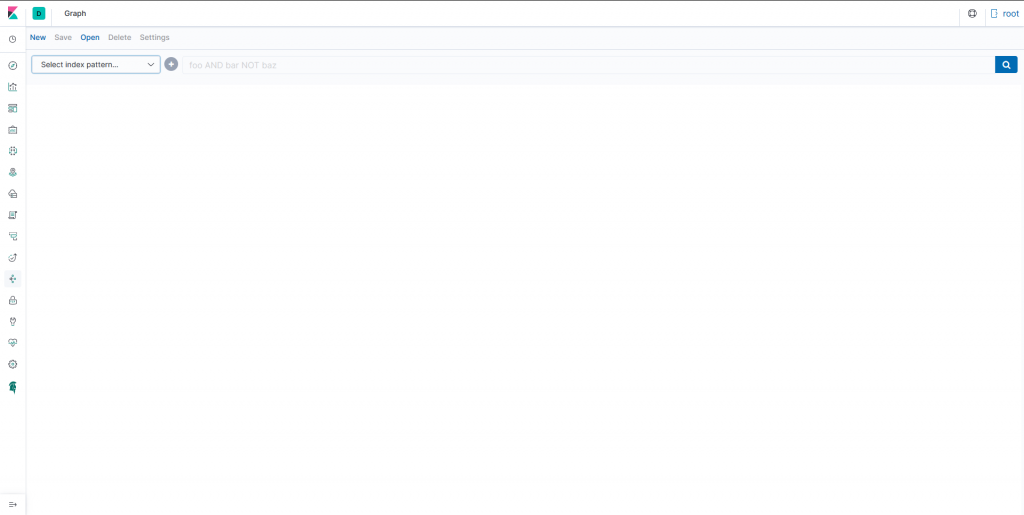The image displays a detailed desktop screenshot featuring multiple toolbars and icons. At the very top of the screen, a toolbar includes an icon in the upper left-hand corner, which consists of a pink triangle overlapping with a quarter of a green circle. Adjacent to this is another icon depicting a bold black letter "D" inside a teal green box, followed by the word "Graph" in white text stretching to the opposite corner, where a globe symbol and a rectangle with the word "root" next to it are located.

Directly beneath this top toolbar is a secondary toolbar with options labeled "New," "Save," "Open," "Delete," and "Settings." The "New" and "Open" buttons are highlighted in blue, while the "Save," "Delete," and "Settings" buttons are grayed out, indicating they are currently inactive.

Below this secondary toolbar is a search or drop-down menu that prompts the selection of an index pattern, displaying the text "select index pattern." To the right of this menu is a circle with a white plus sign, and a grayed-out box containing the text "foo and bar not baz," followed by a search button on the far right.

On the left side of the screen, a vertical toolbar features a variety of icons resembling editing tools. These icons include, from top to bottom, a Roman soldier, a padlock, a small house, a curved arrow, and a wrench.

Overall, the screenshot showcases a complex user interface with multiple layers of functionality and tools, each represented by distinctive icons and text.